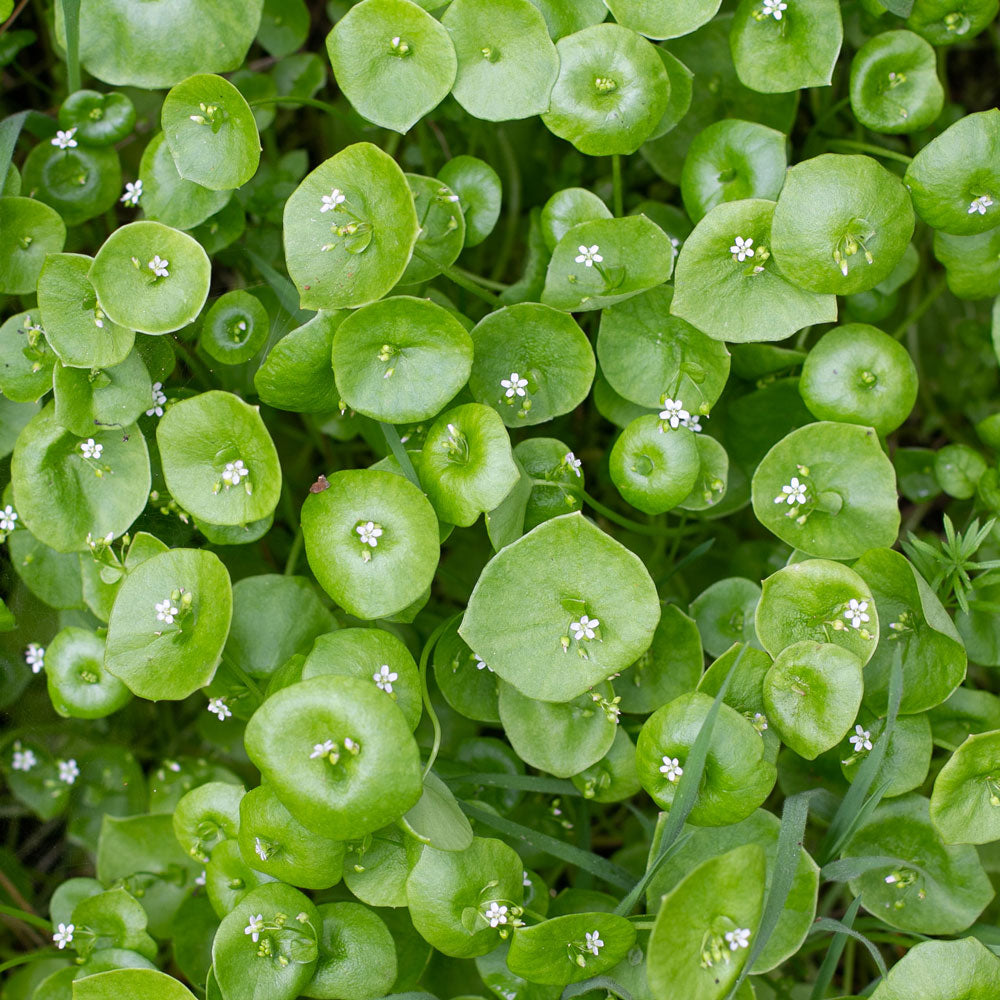This close-up square photograph showcases a lush, dense patch of minor lettuce (Claytonia perfoliata), a vibrant ground cover plant. The plant is characterized by its almost circular, lily pad-shaped leaves that boast a bright, lime green hue with a glossy, waxy appearance. Each of these hardy, flat leaves cradles a delicate, white five-petaled flower at its center, reminiscent of tiny daisies. Interspersed among the minor lettuce, strands of grass subtly weave through the scene, along with a hint of a spiky plant near the center right of the image. Predominantly, the photograph captures the verdant expanse of these young and edible leafy greens, arranged in a natural, almost whimsical pattern, highlighting the detailed, interconnected structure of stems, leaves, and flowers.